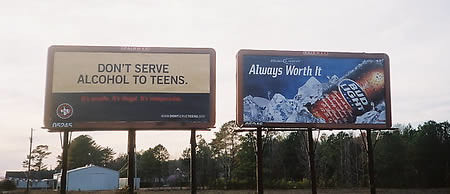Under a gray, overcast sky, a billboard on the left bears the message "Don't Serve Alcohol to Teens," accompanied by a small white square at the top. Below this square, there's an area dominated by white that extends to the bottom right of the image. Within this section are intricate white symbols and patterns on a brown background, which seem to depict the legs of a figure.

The scenery features lush green trees reaching down to the bottom of the image and a barn is nestled in the bottom left corner. 

On the right side of the image, an advertisement depicting a Bud Light beer bottle catches the eye. The label on the brown bottle features a prominent blue circle with the brand name "Bud Light" printed in white text. Below, there's some cursive writing, adding a subtle, ornate detail to the label. The bottle is set against a backdrop suggesting a refreshing, icy environment with ice scattered around.

Overall, the juxtaposition of these elements create a visually rich and engaging scene.